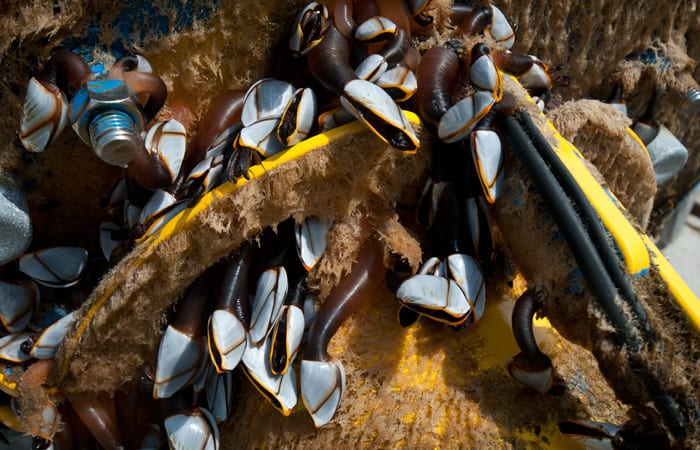This photograph showcases a scene by the shore where a collection of sea creatures, potentially marine worms or insects with a worm-like appearance, have overtaken a man-made object. The image prominently features multiple dark amber-brown, tentacle-like organisms, each ending in bivalve flaps that are gray with thin brown lines. These bivalve flaps, or shells, open and close around their respective tentacles. 

The man-made object, partially visible beneath a layer of fibrous seaweed, includes elements such as yellow plastic parts, rubber pipes, and even the threaded mouth of a water bottle, suggesting significant human debris entangled with the marine life. Additionally, one of the tentacle-like creatures is seen wrapping around a bolt. The background is dominated by a wall of more fibrous seaweed, adding texture to the scene. The overall colors of the photograph skew towards earthy tones with shades of brown and yellow, creating a stark contrast between the natural and the artificial elements within the image.